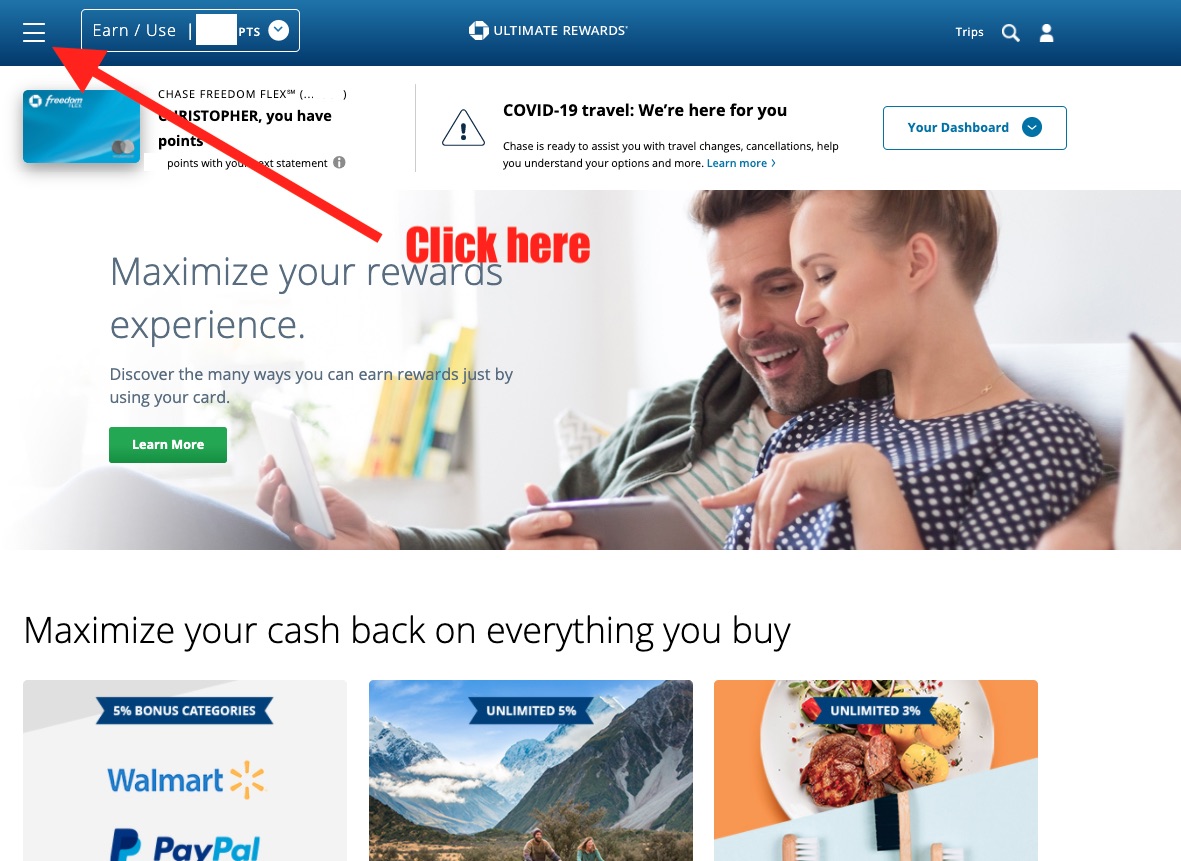The image portrays a promotional webpage likely for a credit card under the "Ultimate Rewards" program. Dominating the top middle of the image is the headline "Ultimate Rewards" in white text, accompanied by a circular logo to its left. The top left corner features three horizontal bars on a blue background extending across the top, highlighted by a red arrow pointing at the bars from the image center. Next to this arrow, red text reads "Click Here."

Centrally positioned within a rectangular frame are two individuals, a man and a woman, who draw immediate attention. The woman, with light brown hair tied up, wears a black blouse adorned with white polka dots and a gold necklace. The man beside her sports a black beard and is dressed in a green sweater over a white shirt with green stripes. He holds a white device, likely a phone or tablet, which both are intently examining. 

At the bottom of the image, there are three square icons. The first icon on the left displays the logos of Walmart and PayPal. The middle icon features scenic images of mountains, evoking a sense of travel or adventure. The rightmost icon depicts an assortment of food items and brushes, suggesting themes of culinary or artistic rewards.